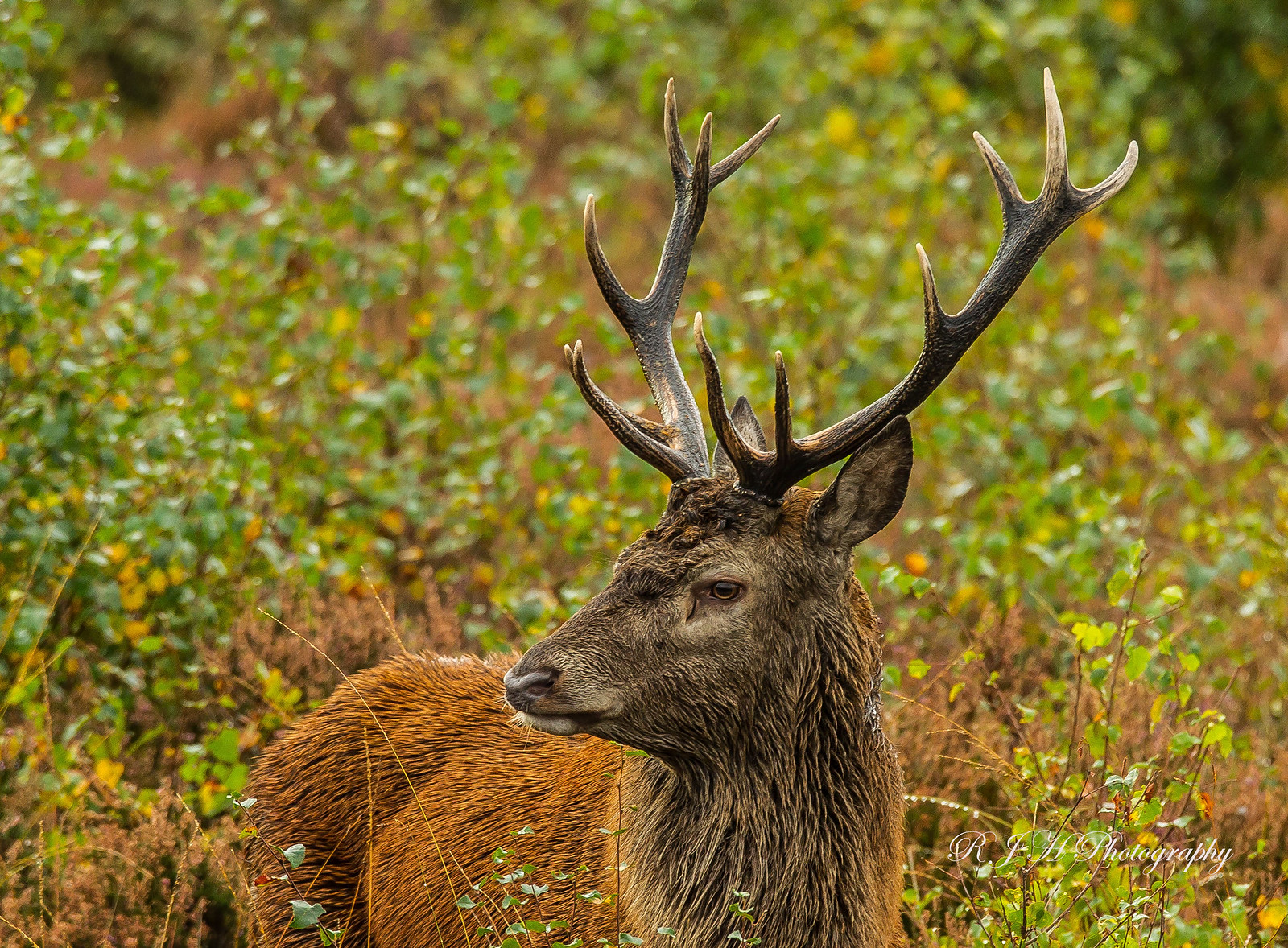In this image, we see a vivid nature scene set during the day, with a backdrop of small leaves and bushes that are currently in transition, displaying a mix of greens and yellows, accompanied by some dead brush. The background appears somewhat blurry, enhancing the focus on the main subject in the foreground.

Dominating the foreground is a male deer, likely an elk, standing close to the camera. The animal displays a striking set of antlers, each bearing approximately six distinct smaller horns, reaching a medium height with three tiers high and slightly wider than its head. The deer's body is tilted towards the 5 o'clock position, while its head, characterized by a darker brown neck, is turned towards the 7 o'clock position, gazing intently at the observer with its eye visible.

The deer’s coat transitions from the dark brown of its neck and head to a reddish brown along its body and hindquarters, blending seamlessly with the background of mixed green and reddish-brown foliage. The antlers stand out with their deep brown to black colors, subtly highlighted by whitish tips, creating a harmonious contrast with the natural setting, which adds a dynamic visual complexity to the scene.